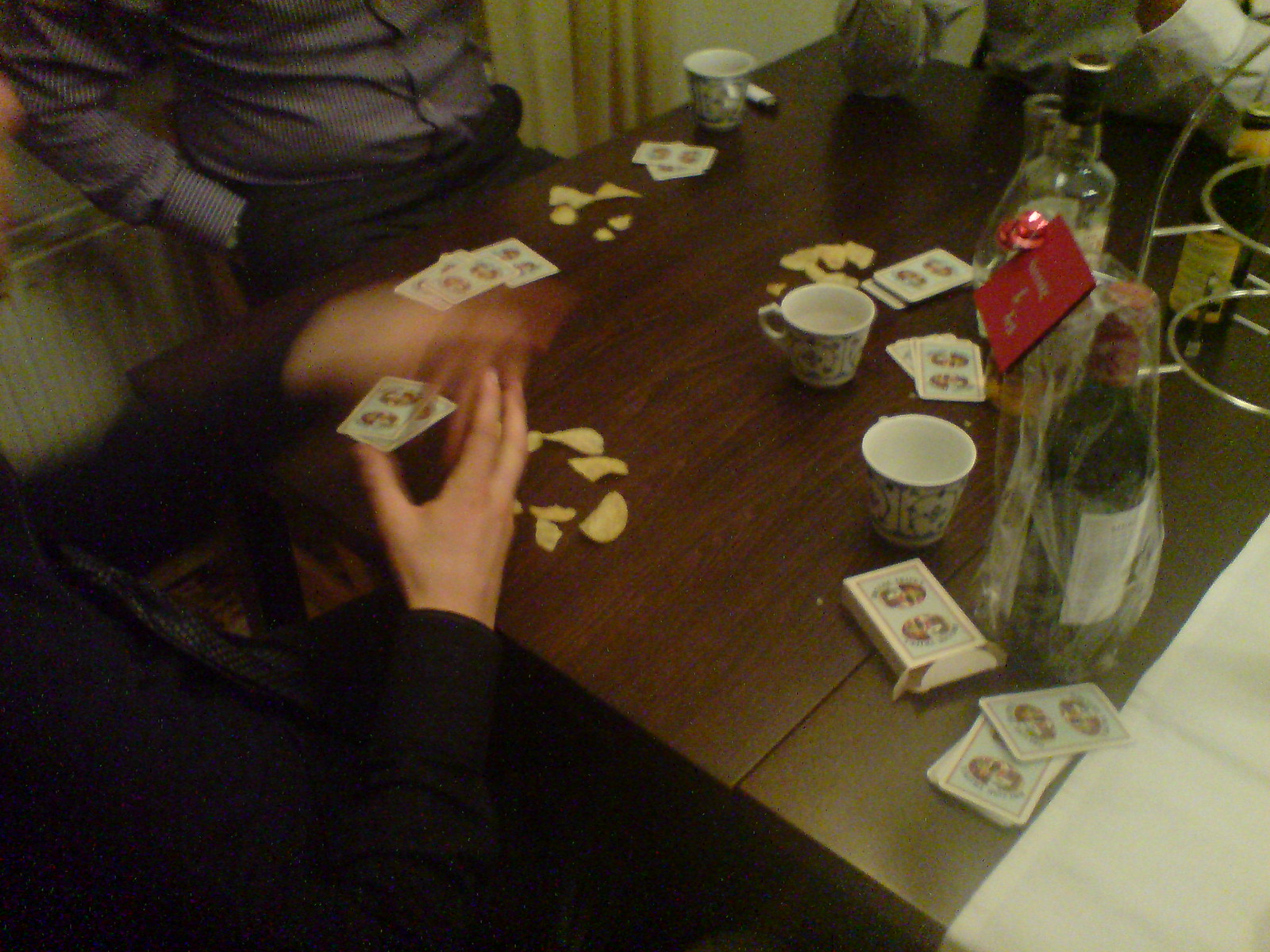This photograph depicts an intriguing scene of a card game in progress at a cluttered wooden table. Various bottles, glasses, and cups are scattered across the surface, suggesting that the players might be enjoying a lively evening. On the far left, a man dressed in black has his back to the camera. His left hand is visible but slightly out of focus, while his right hand is moving so swiftly that it appears as a blur, hinting at rapid shuffling or some other quick hand motion.

To his left, another man, clad in a gray long-sleeve shirt and black pants, sits with his hands conspicuously tucked into his pockets, an unusual posture for a card player. Across the table, only the forearms and a small portion of the chest of a third player are visible. This individual, also wearing a gray long-sleeve shirt, contributes to the paradoxical nature of the scene.

The table is strewn with playing cards, yet the players appear to be wagering with potato chips, an odd choice unless these chips hold some unconventional value. The combination of the man's unnaturally fast-moving hand and the strange betting items creates an overall sense of surrealism and intrigue in what would otherwise be a mundane card game.